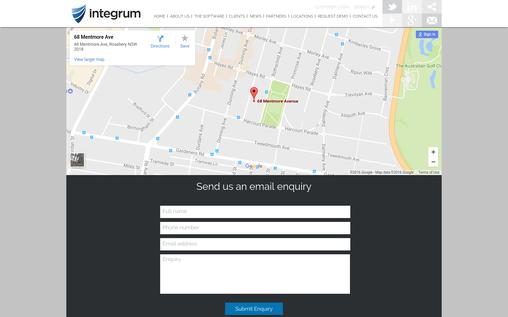Here's a cleaned-up and detailed caption for the image:

---

A screenshot from an interactive map on a website named "INTEGRAM" features a detailed layout with various elements. The map is highlighted with a white outline and contains bands of blue shades—light blue, mid blue, and dark blue—indicating different regions or layers. The top navigation bar displays clickable tabs labeled "Home," "About Us," and several other sections, culminating in a "Contact Us" tab. These sections are separated with faded text.

On the left of the map, there are faintly visible gray squares featuring social media icons. The first dark gray square depicts a white bird for Twitter (or X). Next, a lighter gray square with the letters "I" and "N" represents Instagram. A mid-gray square with an icon of three connected squares suggests a sharing function. Another similar square with a white circle might indicate LinkedIn, followed by another gray square with a white "G" for Google. Lastly, a dark gray square with a frowny face icon stands unclear in its association.

The map itself is detailed with Google Maps elements, including gray and tan depictions of roads and buildings, accompanied by red location pins. To the far right, green patches of grass and blue water bodies are visible. A white pop-up rectangle on the left side contains the address "68 Murdroe Avenue" in black text. There is some heavily blurred black text underneath, along with a blue hyperlinked text probably reading "View Larger Map."

On the right side of the map, there are navigation arrows—a gray one pointing left and a dark blue one pointing right—indicating direction. Beneath these arrows, "Directions" is written in bold blue text, alongside a gray star with "Save" in blue hyperlink text below it. 

Towards the bottom of the screen, a large black bordered rectangle contains the call-to-action "Send Us an Email Inquiry" in dark gray text. Several input fields are aligned vertically: the first three small rectangles are labeled "Full Name," "Phone Number," and "Email Address" respectively. The last input field is larger but its label is too blurred to read. At the bottom of this section, a dark blue rectangle with thin white text displays "Submit Inquiry," though misspelled as "ENQUARY."

---